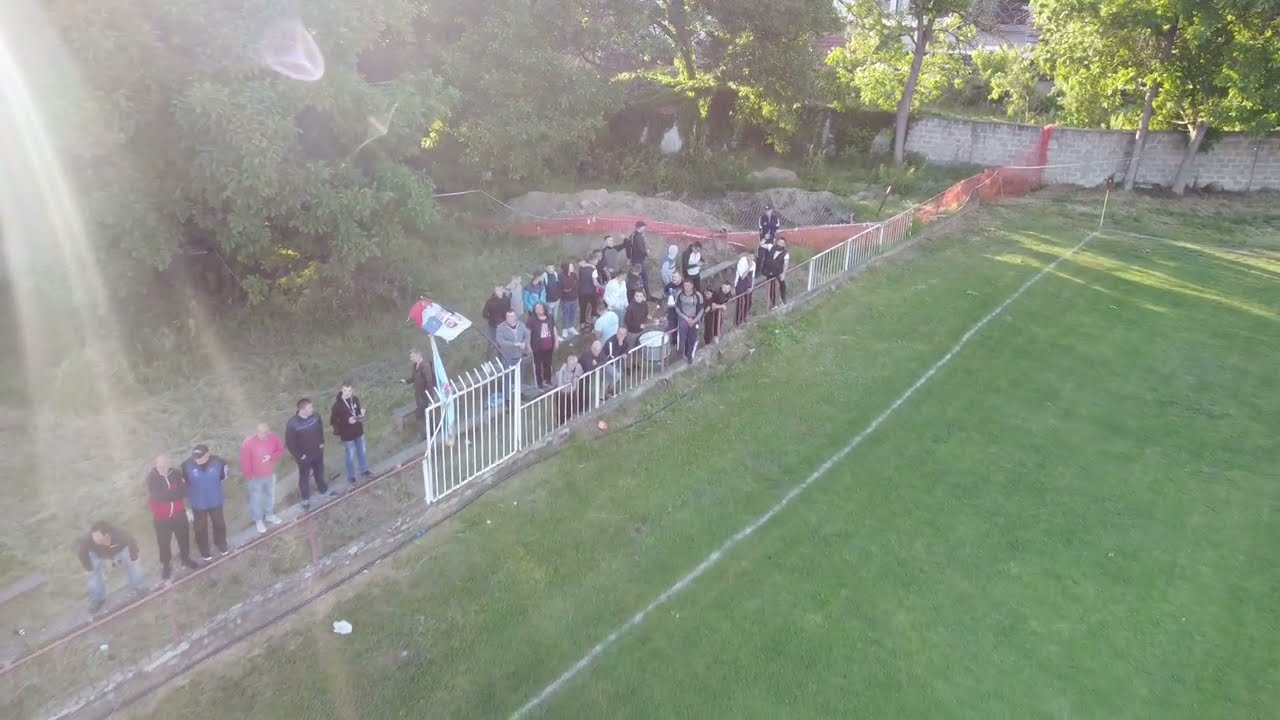This aerial, somewhat downward-angled photograph showcases a sports field bathed in bright sunlight filtering from the top left corner to almost the bottom of the image. A distinct white line, likely made of lime, runs diagonally across the field near the center. To the left of this line, a partially rusted white gate and chain-link fence stretches from the bottom left to near the top right of the frame. Behind this fence on the left, a group of approximately 20 spectators, dressed primarily in black shirts and jeans, stand in a somewhat orderly line, facing towards the right. Behind the spectators lies more grass, leading to a backdrop of tree leaves and a short stone wall partially covered with vines from which more trees emerge, marking the top right and center of the image.